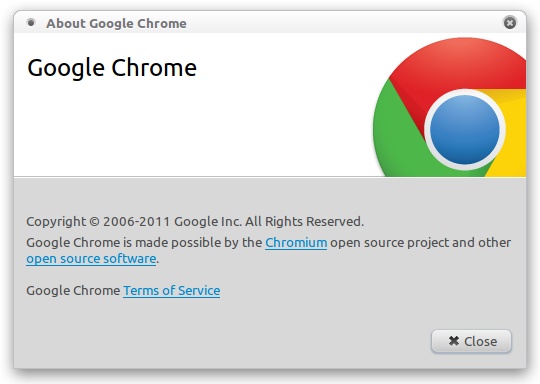The image illustrates the "About Google Chrome" screen, providing a detailed overview of the browser's information. At the very top, the title "About Google Chrome" is prominently displayed. Below this header lies a large white rectangle featuring the name "Google Chrome" in dark lettering. Positioned to the far right within this section is the distinctive Google logo: a central blue circle encircled by a white ring, with outward swirling segments in red, yellow, and green.

Beneath this white section is a gray box containing textual information. It states "Copyright 2006-2011, Google Inc. All Rights Reserved. Google Chrome is made possible by the Chromium Open Source Project and other open source software." The phrases "Chromium Open Source Project" and "open source software" are highlighted in blue, suggesting they are clickable hyperlinks. Furthermore, the text "Google Chrome, Terms of Service" also appears, with "Terms of Service" in blue, indicating it as another hyperlink.

In the bottom right corner of this gray section is a light gray rectangle with a dark "X" and the word "Close," which serves as a button to exit the "About" screen.